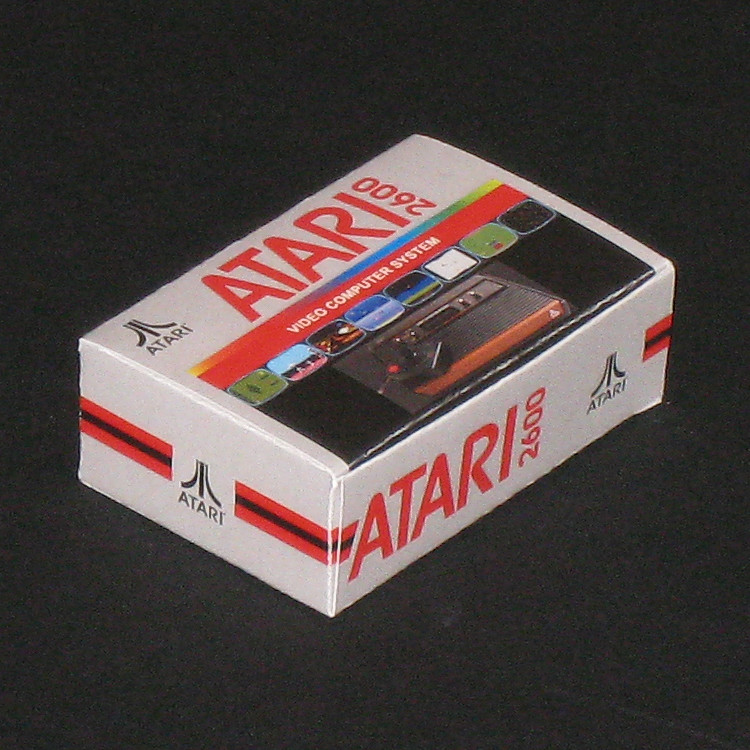Here is the cleaned-up and detailed caption for the image:

"An angled view of an old Atari 2600 box, displaying two sides and the top. The box is primarily a whitish-gray color with several 'Atari' logos prominently featured. On both visible sides, 'Atari' is written in bold red letters along with '2600.' The end side shows 'Atari' in black. The top surface features 'Atari' in black in the left-hand corner and again in red across the middle, also including '2600.' A weathered image of the Atari 2600 console and its joystick controller takes up the lower section of the top surface, with 'Video Computer System' printed above it along with various icons. The box shows clear signs of aging, with noticeable wear on the corners and faded black sections, reflecting its vintage status."